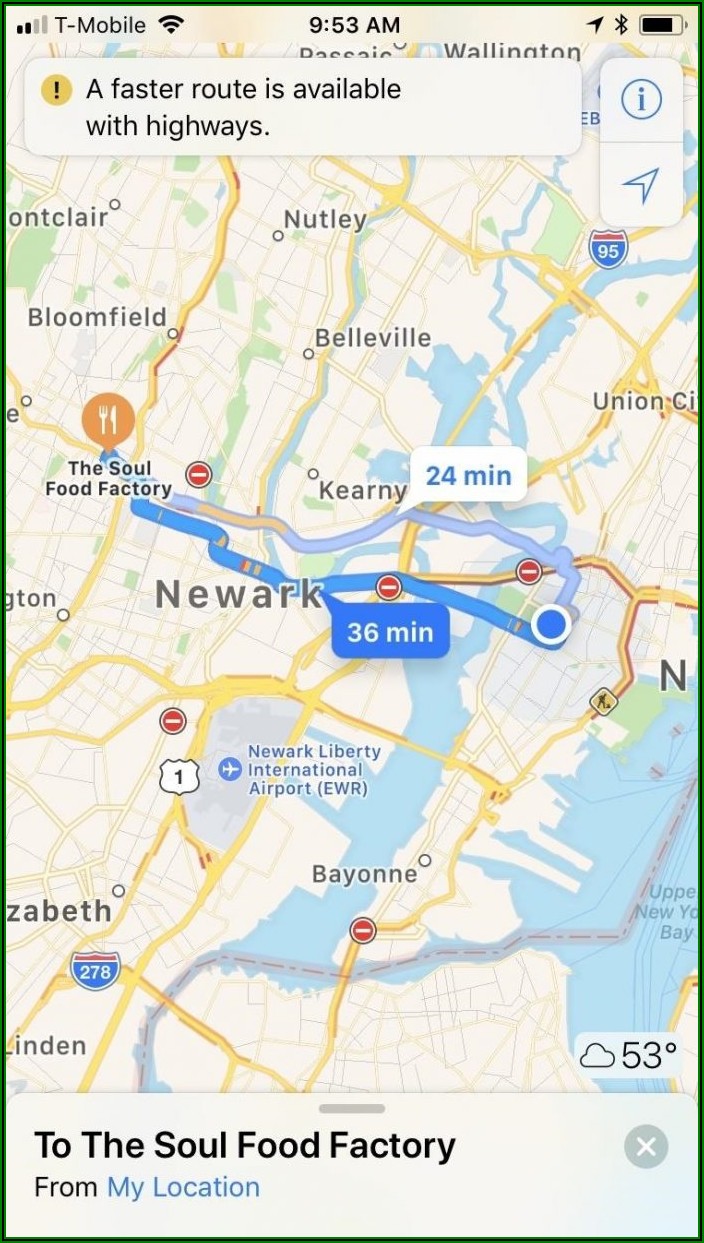A detailed and clean caption for the provided image could be:

"Screenshot of a cell phone displaying a GPS navigation app. The main background is a map highlighting a route with estimated travel times of 36 minutes in one direction and 24 minutes in the reverse. The destination marked on the map is 'Soul Food Factory,' originating 'From My Location' as indicated in a white bar at the bottom, next to an 'X' circle on the right. The map also shows various cities, including Notley, Belleville, and Bloomfield, with Newark prominently centered. Key landmarks such as the Newark Liberty International Airport and the Soul Food Factory are clearly labeled. The time displayed on the phone is 9:53 AM."